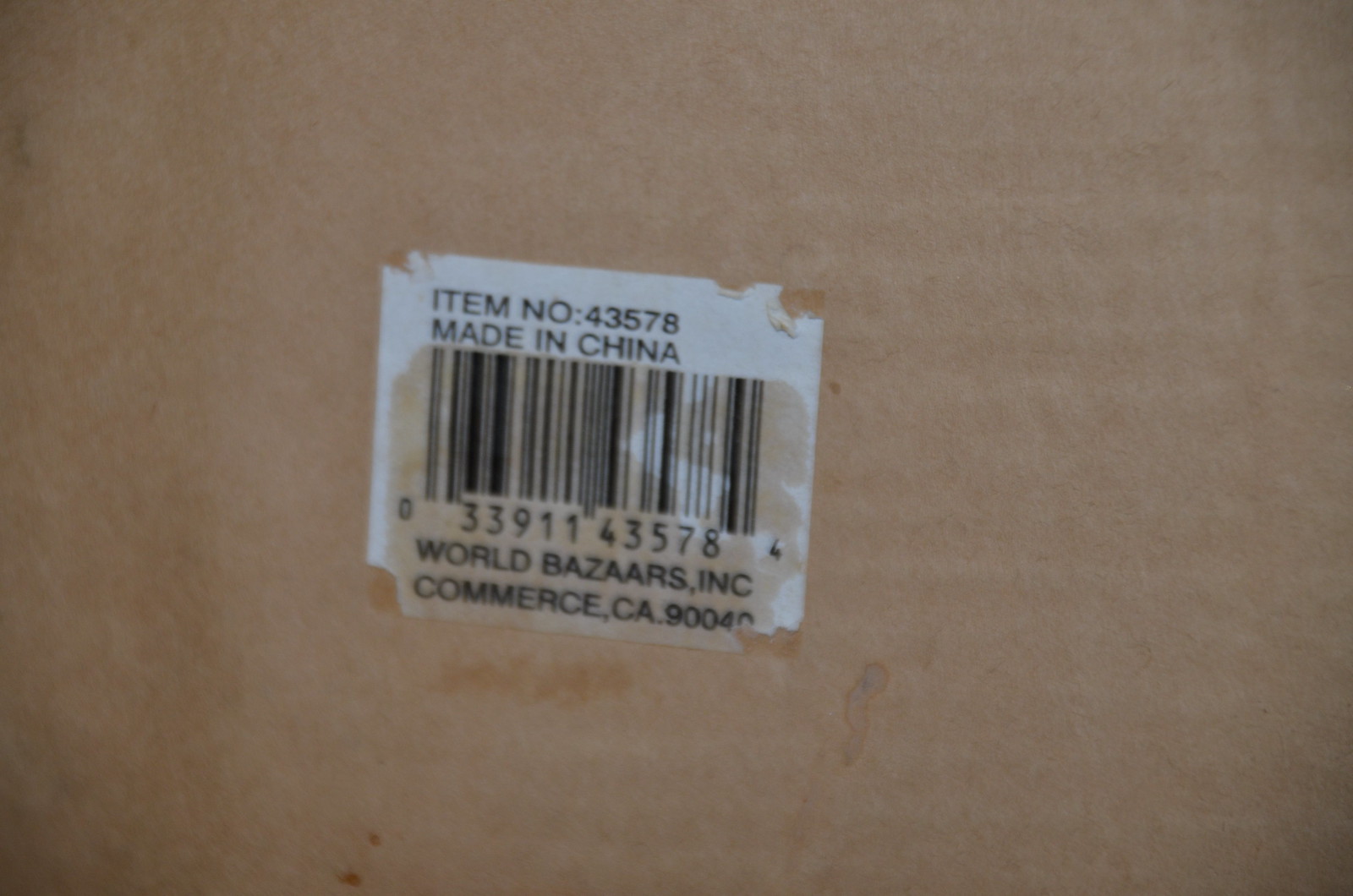The image depicts a close-up shot of the back of an unidentified product, prominently featuring a sticky price tag. The background, which could be either a wall or cardboard due to its brown color, serves as an unidentifiable surface onto which the price tag is adhered. The tag itself reads:

- Item Number: 43578
- Made in China
- Barcode
- World Bazaars Inc., Commerce, California 90040

The tag appears slightly damp, resulting in some smearing of the printed numbers.